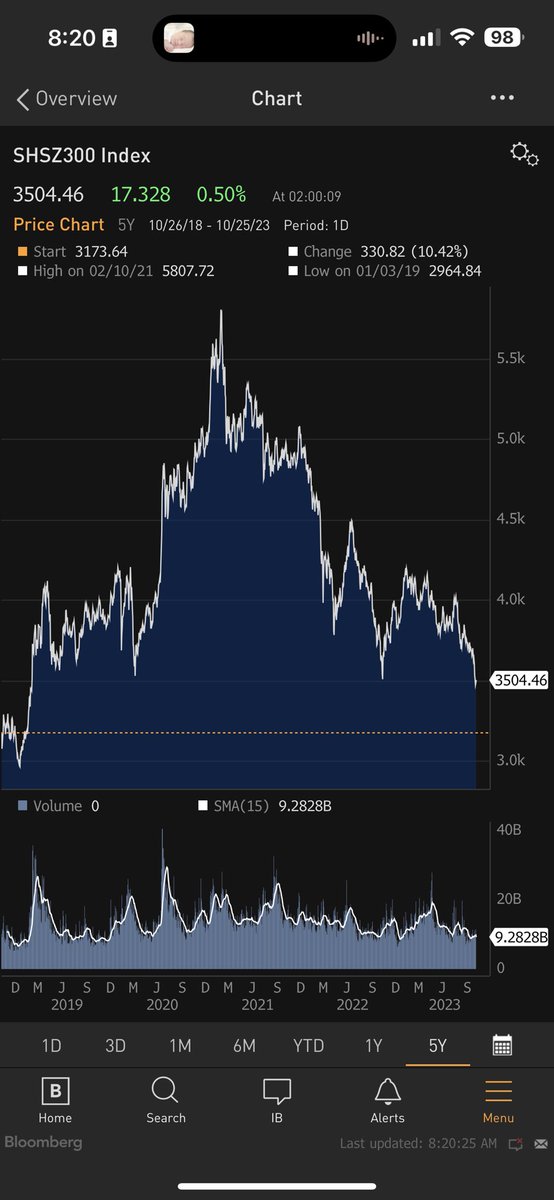This image is a screenshot from the Bloomberg app on a smartphone, displaying financial news and data. At the bottom of the screen, there is a navigation bar with icons for Home, Search, IB (messaging), Alerts, and Menu, confirming that it's indeed the Bloomberg app. Just above the navigation bar, the Bloomberg logo, a square with a 'B' in it, is visible. 

The main focus of the screenshot is a detailed price chart of the SHSZ 300 index, which spans from values as low as 3,000 to as high as 5,500. The chart highlights a peak in the middle of the timeframe, where the index value exceeds 5,500, potentially approaching 6,000. Below this, there's another, smaller graph covering a longer timeframe from 2019 to 2023, providing a more extended overview of the index's performance over these years. The screenshot represents a comprehensive display of financial data, typical of Bloomberg's detailed analysis and news coverage.